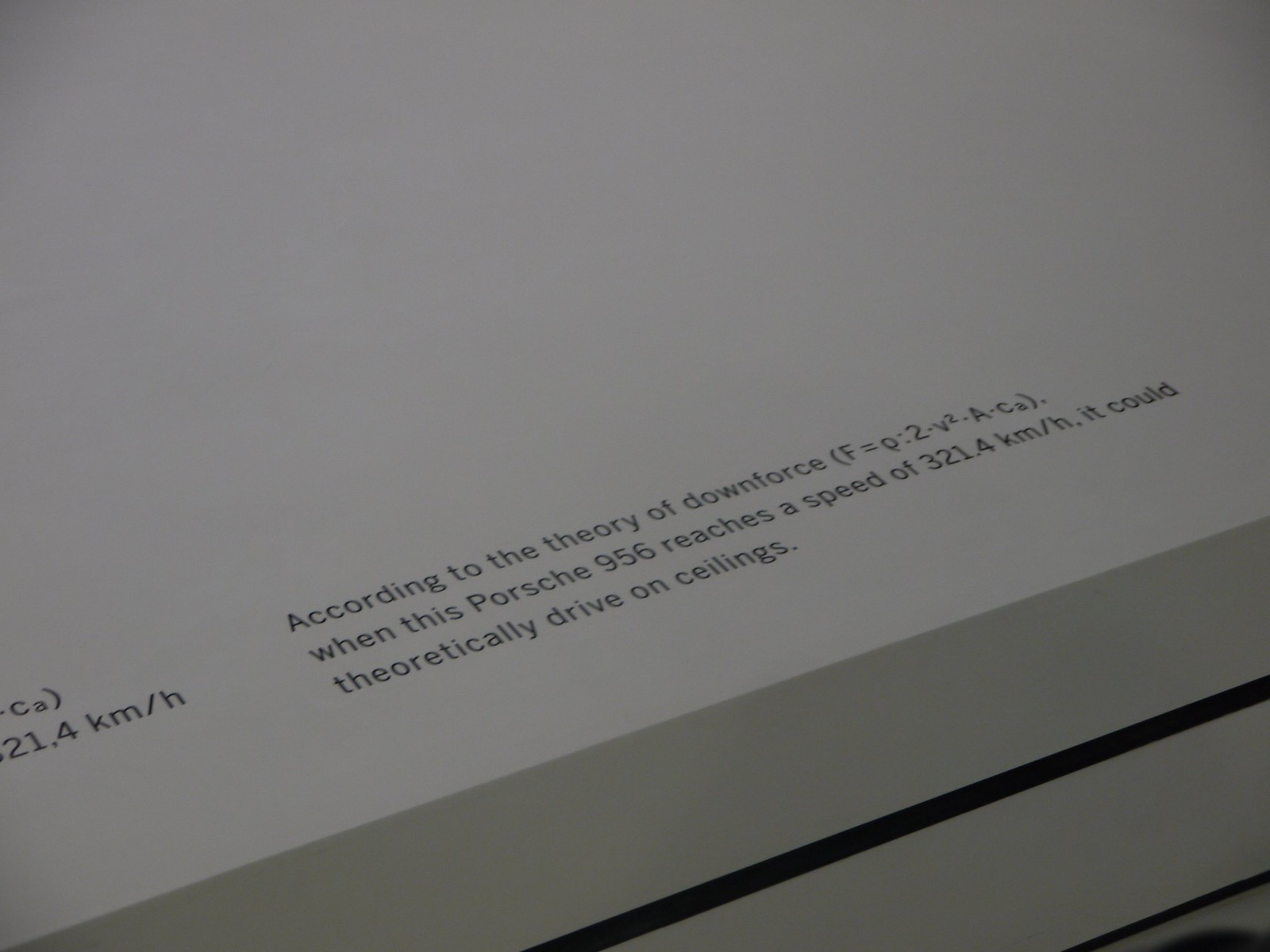The image depicts an extreme close-up of a surface, resembling either a part of a high-tech machine such as a printer or possibly the hood of a Porsche 956. The background is primarily white with a series of black and white lines creating a geometric pattern, notably the thick white lines and thinner black lines near the bottom right corner. Prominently featured is black text that partially describes the theory of downforce, including details like "CA (21.4 KM/H) according to the theory of downforce F (F=Q2V2ACA)," indicating that when the Porsche 956 reaches a speed of 321.4 kilometers per hour, it theoretically possesses enough downforce to drive on ceilings. The text, although fragmented, emphasizes the scientific calculation behind the car's potential aerodynamic performance. The close-up nature of the image obscures other identifying features, making it challenging to confirm whether it is indeed a car or another object.